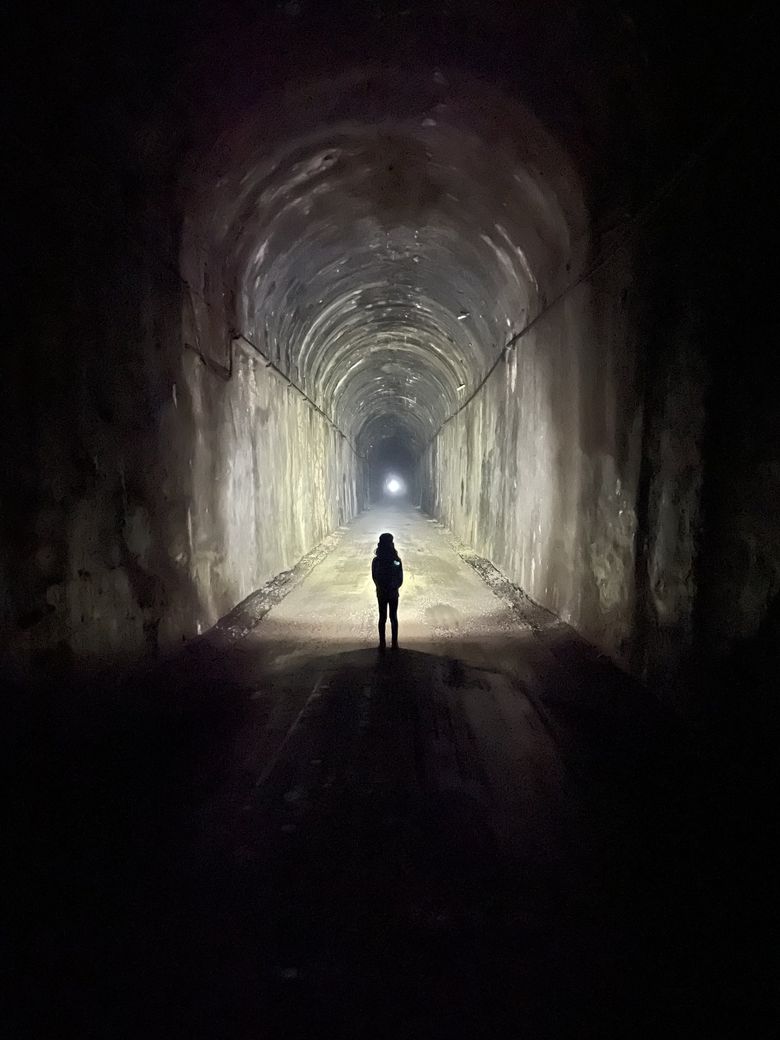This artwork, taller than it is wide, portrays the dark interior of an arched tunnel with aged, discolored walls and a stained floor, suggesting its construction from concrete or stone. The tunnel's narrow width, roughly 10 to 12 feet, and its tall arched ceiling present an imposing frame. The predominant beige tones on the walls, floor, and ceiling transition to darker shades near the top. Toward the middle of the image but positioned within the front half of the tunnel stands a petite, shadowy silhouette of a figure, possibly a child or a female, facing the light. The figure's hands, indistinctly shown, may be in their pockets or crossed. The far end of the tunnel features a small, stark white light against a solid black background, casting an eerie glow that partially illuminates the tunnel's interior. The surrounding edges of the painting are enveloped in darkness, intensifying the contrast between the tunnel and the pitch-black area outside. The overall atmosphere is one of neglect and decay, hinting at a long-forgotten desolation.